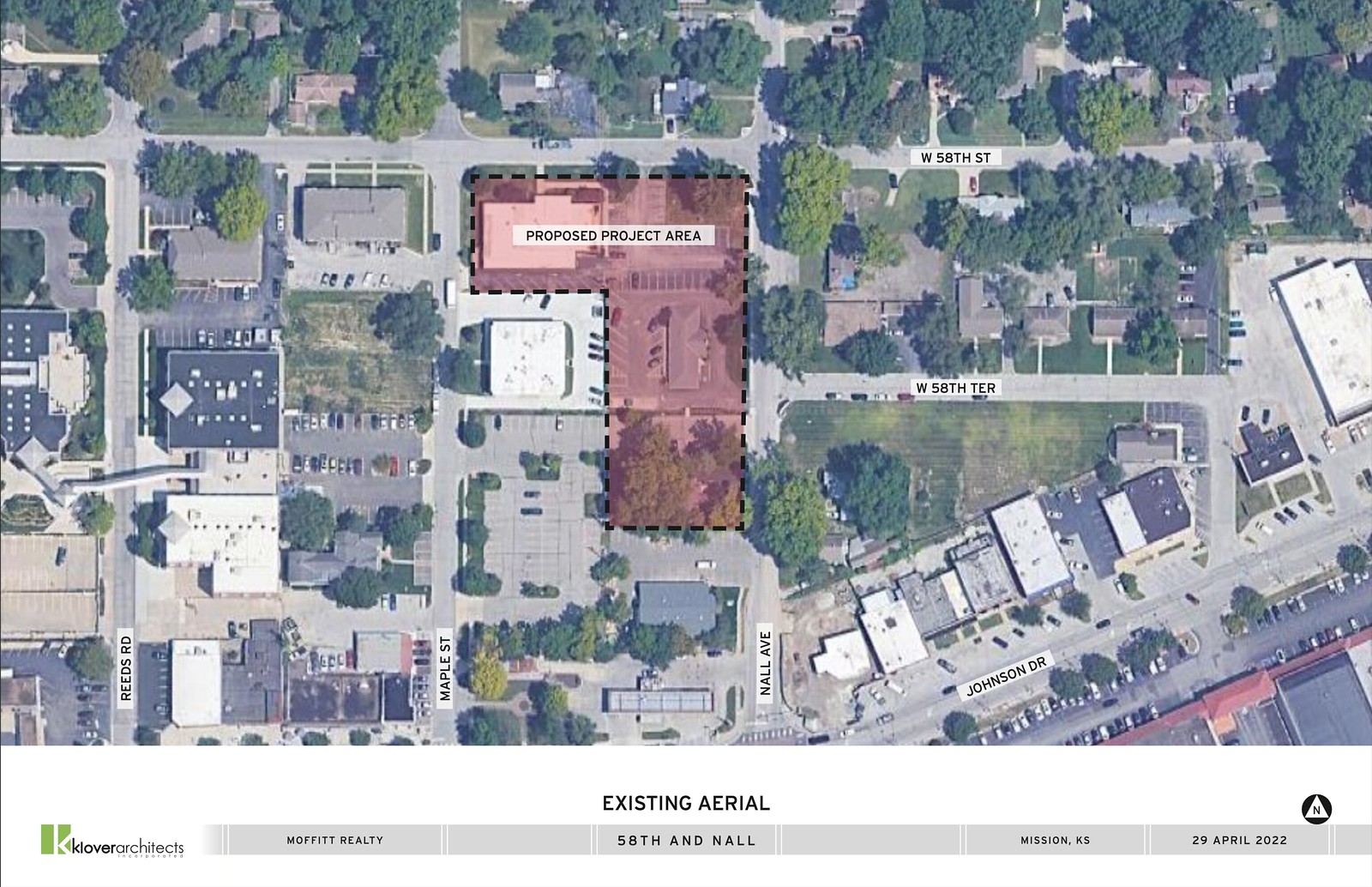This image provides a detailed aerial view of a city, showcasing an area highlighted in light red with a dashed black outline, resembling an upside-down L shape. Within this highlighted section, which is labeled "Proposed Project Area," multiple buildings are visible both inside and outside the boundary. Towards the left side of the image, there is a parked car in a parking lot situated on the right side of the road. The text "Existing Aerial" is displayed at the bottom of the image, accompanied by a logo for Clover Architects featuring a green rectangle with the letter 'K' inside. Below the image, a gray bar contains the text, "Moffett Realty, 58th and Nall, Mission, Kansas, 29 April 2022."